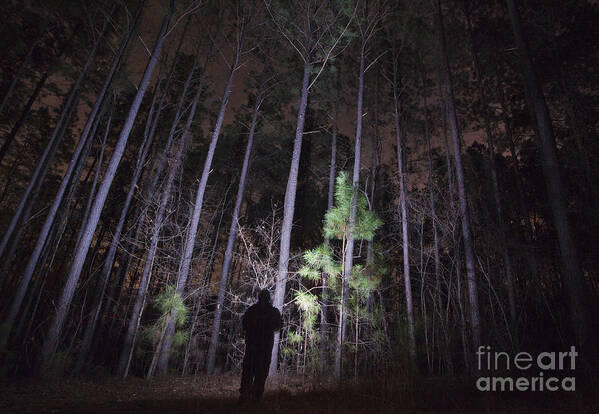The image captures a dense forest at night with an eerie, dark pink sky. At the center stands a silhouetted man, holding a bright flashlight that starkly illuminates the immediate area around him. The forest is filled with very tall, thin trees, primarily pines, their trunks a ghostly gray and their needles a shimmering green in the light. These trees soar well above 30-40 feet into the air, blending into the dark, smoky sky. The light creates a stark contrast, with the trees directly in front brightly illuminated, while the ones further away fade into shadow. The forest floor is littered with fallen leaves, adding to the nocturnal mystery. In the lower right corner, a watermark reads "Fine Art America" in light gray text, adding a subtle touch of authenticity to the artwork.